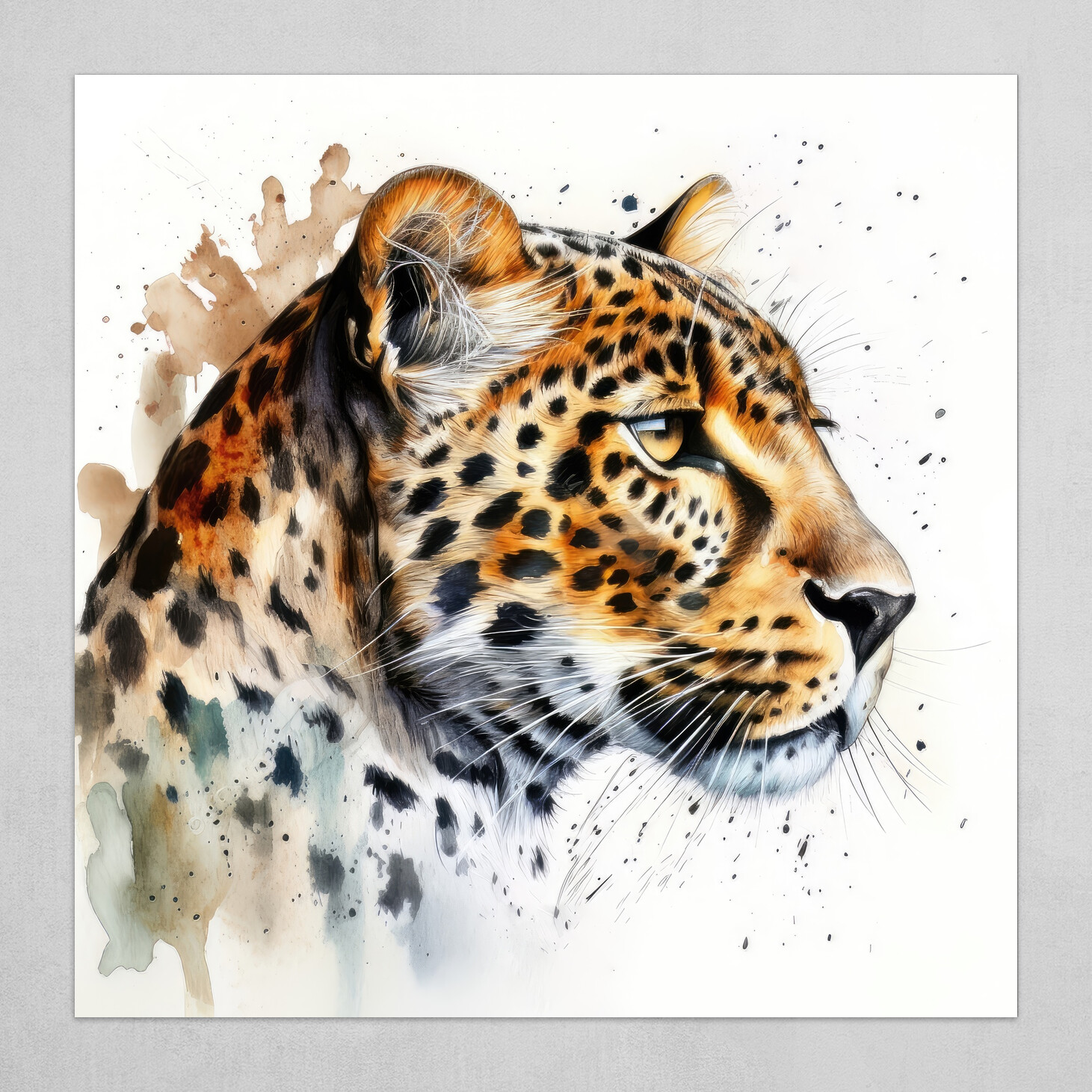This detailed watercolor painting features the head of a cheetah, meticulously rendered with vibrant orange, white, and black hues. The focal point of the artwork is the cheetah's face, depicted with an exquisite level of detail that highlights its distinctive black spots and the fine hairs emerging from its ears. The eyes, a captivating golden amber, reflect light, adding a lifelike quality and depth to the piece. The cheetah is portrayed from a side profile, gazing contemplatively into the distance. The background is predominantly white with expressive splashes of orange and flecks of black, enhancing the dynamic composition. The entire image is bordered by a gray frame, which compensates the vivid colors of the cheetah and provides a polished finish to the overall presentation.